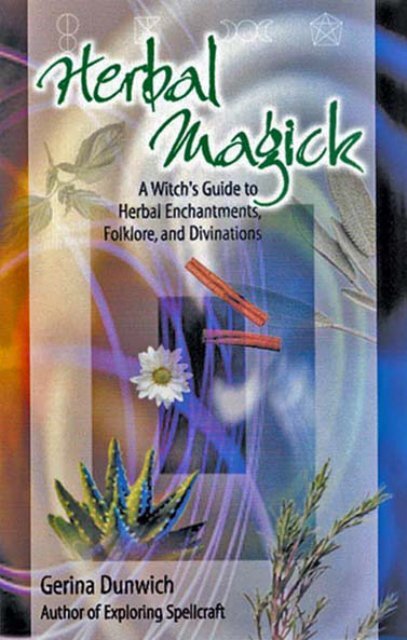The cover of the book titled *Herbal Magick: A Witch's Guide to Herbal Enchantments, Folklore, and Divinations* by Gerina Dunwich—renowned author of *Exploring Spellcraft*—features a nostalgic early 2000s graphic design. The title is elegantly set in green italic script at the top, while a blocky black text below it details the subtitle. The author's name appears in the bottom left corner, in a similar typeset. The background is a swirling, mystical collage of blue, purple, yellow, orange, and pastel hues, giving off an aura of enchanting energy.

Overlaying the vibrant background is an array of transparent, clipped images of various herbs. Notable among these are cinnamon sticks, aloe vera, what appears to be a chamomile flower, sage, rosemary, and other greenery, all arranged in a low-quality, almost clip art style. These elements, combined with the colorful, abstract backdrop, evoke a sense of ancient herbal wisdom intertwined with magical folklore.